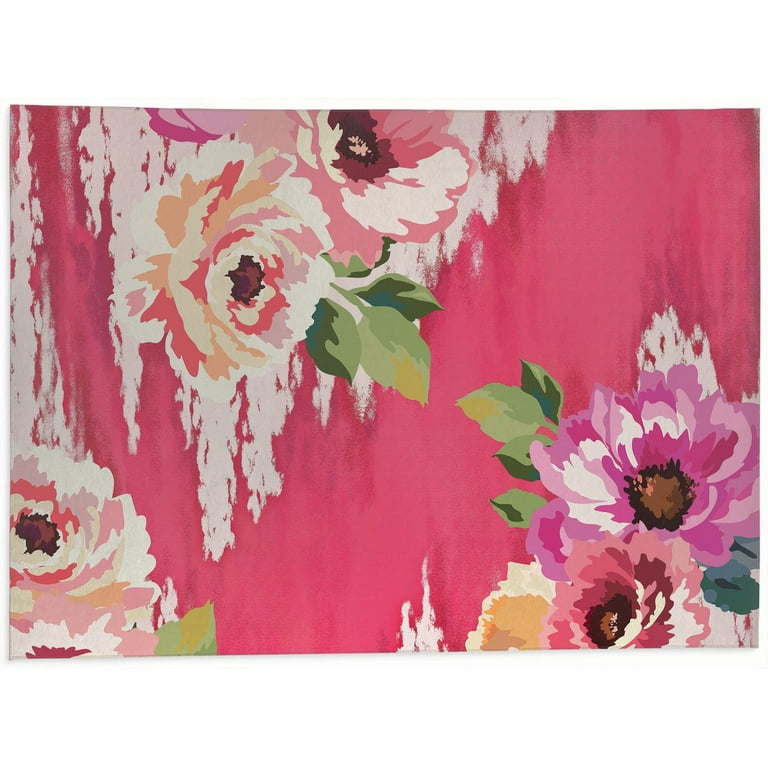The image depicts a vibrant scene that resembles either a painting or fabric, possibly a tapestry or wallpaper. The background is a striking hot pink, occasionally referred to as carnation pink. Scattered across this vivid backdrop are large, colorful flowers painted in various shades, including pink, purple, blue, beige, and white. Apricot and cream-colored blooms add to the rich palette, complemented by burgundy and light pink flowers, creating a diverse and lively floral arrangement. Green leaves in lighter and darker hues intermingle among the flowers, with some white vine-like elements weaving through. The artwork appears to be crafted with watercolor, lending it a soft, almost ethereal quality, and it gives the impression of delicate fabric adorned with an intricate, floral design.